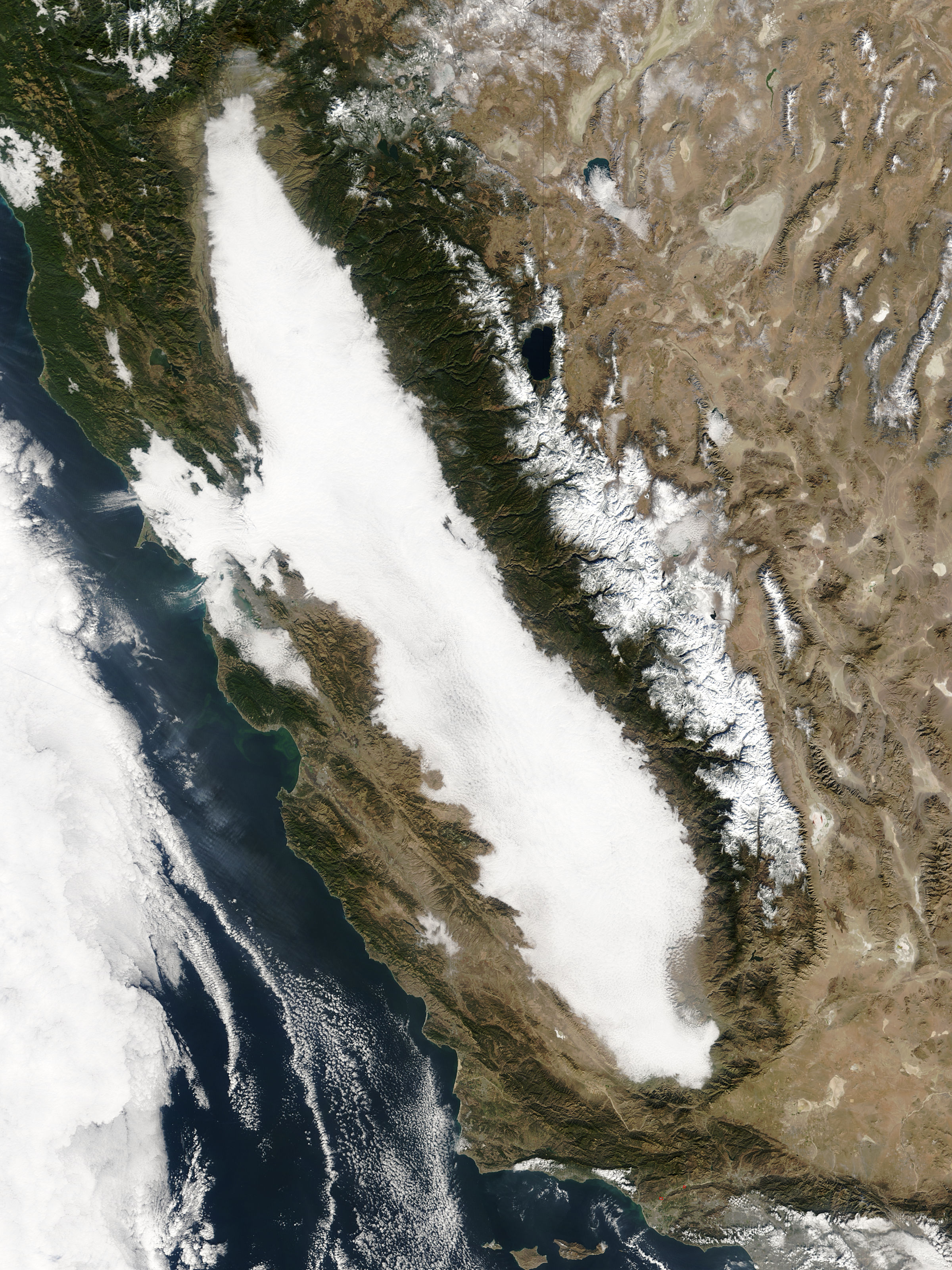The image is a high-altitude photograph, possibly taken from a satellite or an airplane, showing a diverse landscape. In the left-hand corner, the image features a triangular blue area, akin to a body of water, with its vertices positioned as follows: the bottom left corner, an inch down from the top left corner, and an inch to the left from the bottom right corner. Adjacent to this water body, clouds stretch from the top to the bottom of the left side, gradually dissipating as they move rightward. A large triangular landmass occupies the central area, transitioning into a vast, oval-shaped region encircled by rocky terrain and mountains. This oval area is predominantly white, suggesting it is covered in snow. Prominent cliff faces and towering mountains emerge from its borders, leading into a rugged expanse of brown terrain with scattered white spots. The top left portion of the image hints at some green areas, possibly indicating vegetation. Overall, the scene captures a dramatic contrast between aquatic, snowy, and mountainous elements.